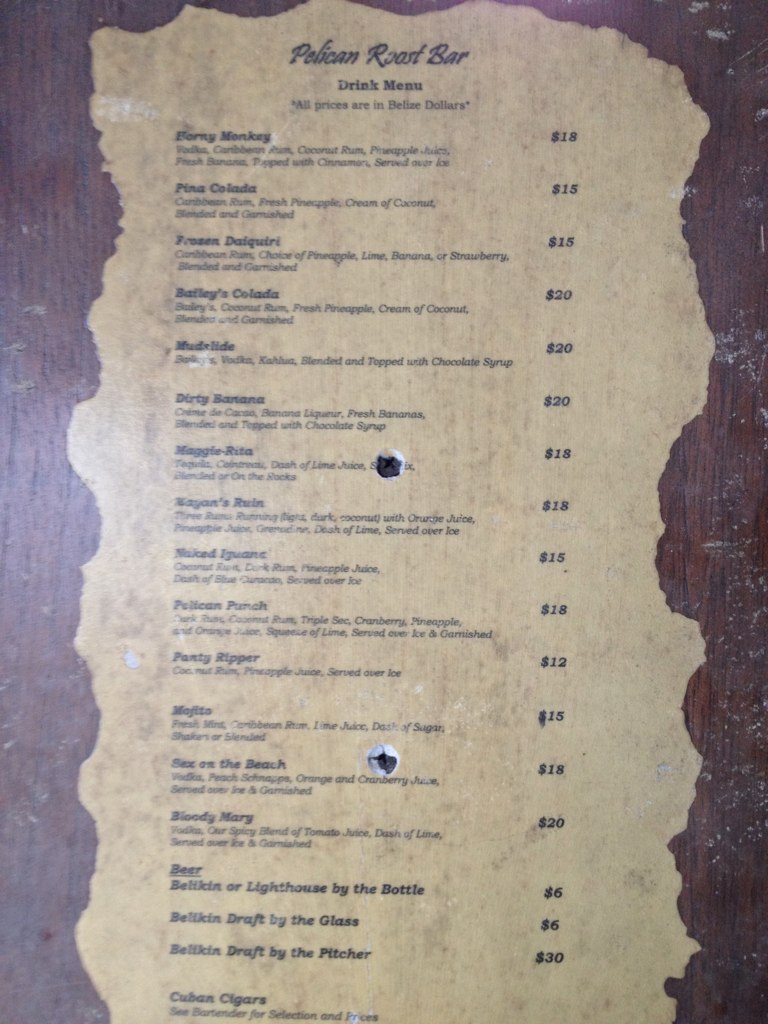This photograph captures a drinks menu affixed to the wall of a drinking establishment, likely a bar. The menu is presented on an off-white, ivory-colored backdrop, intentionally designed with a weathered aesthetic. This central ivory section is outlined by a jagged, torn-style border, giving the impression of a ripped sheet of paper. Surrounding this is a faux wood surface, designed to look like brown laminate with vertically running wood grain patterns. The laminate shows signs of wear, evidenced by lighter gray scuff marks, particularly prominent on the lower left portion where light is reflecting more intensely compared to the upper and right sections.

Two gray Phillips head screws secure the menu to the wall, one positioned roughly at the center and the other slightly lower. The areas around these screws display minor cracking and peeling, with one screw piercing directly through a line of text. 

At the top of the menu, in a handwritten script, is the name "Pelican Road Bar," followed by the bolded title "Drink Menu." Just beneath this, in very small, barely legible print, is the note "All prices are in Belize dollars." The menu features a left-aligned list of drinks, each name bolded, with one to two lines of non-bolded descriptive text underneath. On the right, a column of prices aligns with each drink, ranging from $6 to $30. The careful layout and design details reflect an establishment that values both aesthetics and practical information for its patrons.